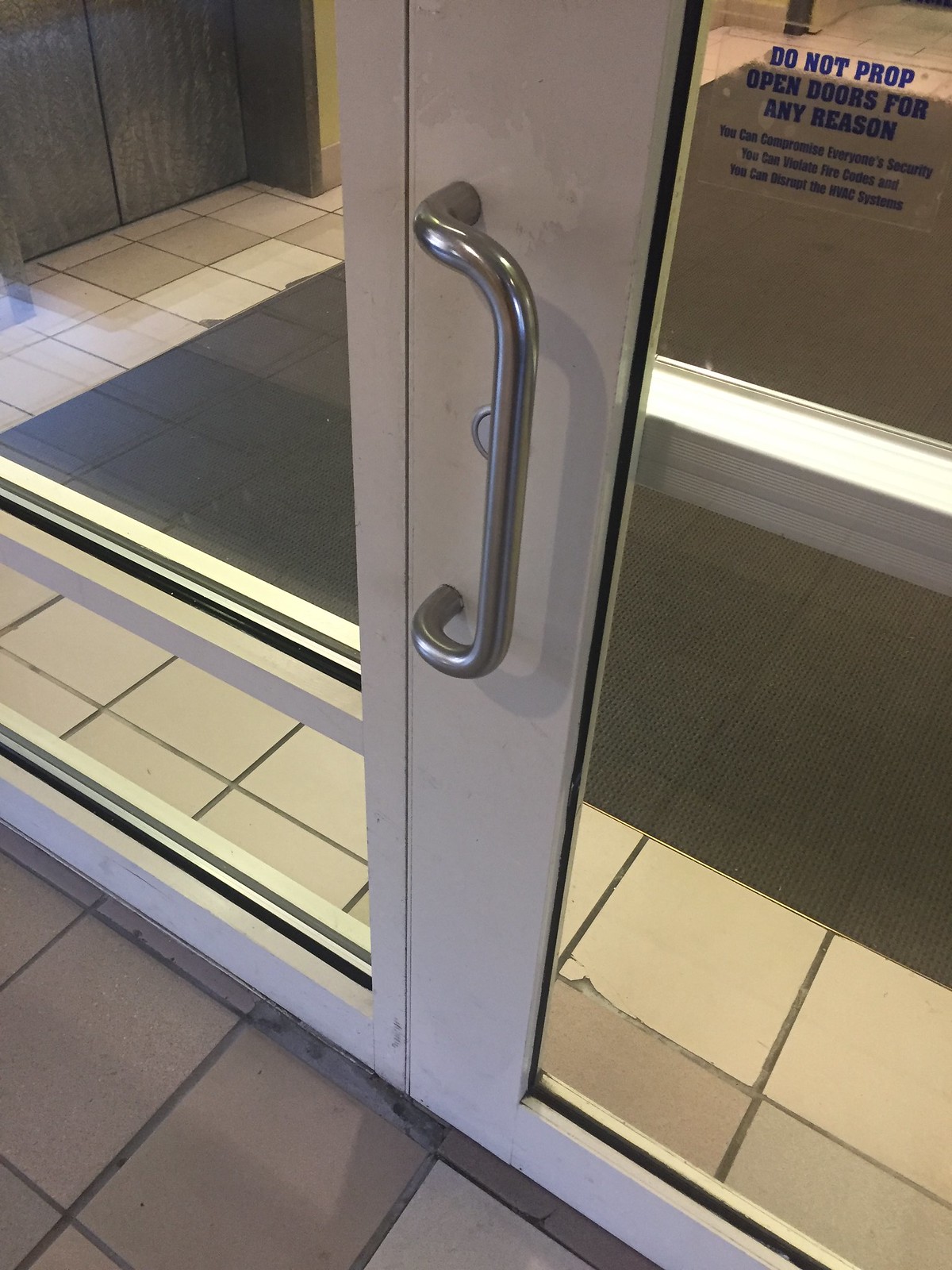The image depicts a metal-framed commercial door with a large glass center. The door features a silver pull handle on the outside and a horizontal push bar inside. Prominently displayed is a sticker stating, “Do not prop open door for any reason,” emphasizing security, fire code compliance, and HVAC system integrity. Through the glass, the interior reveals a white ceramic tile floor, some of which appear cracked, alongside a large black commercial mat. To the upper left, the lower half of brownish-gray elevator doors is visible. Additionally, there is another large glass panel adjacent to the door, offering a clear view into the building. The door frame is finished in beige, blending into the overall commercial ambiance.